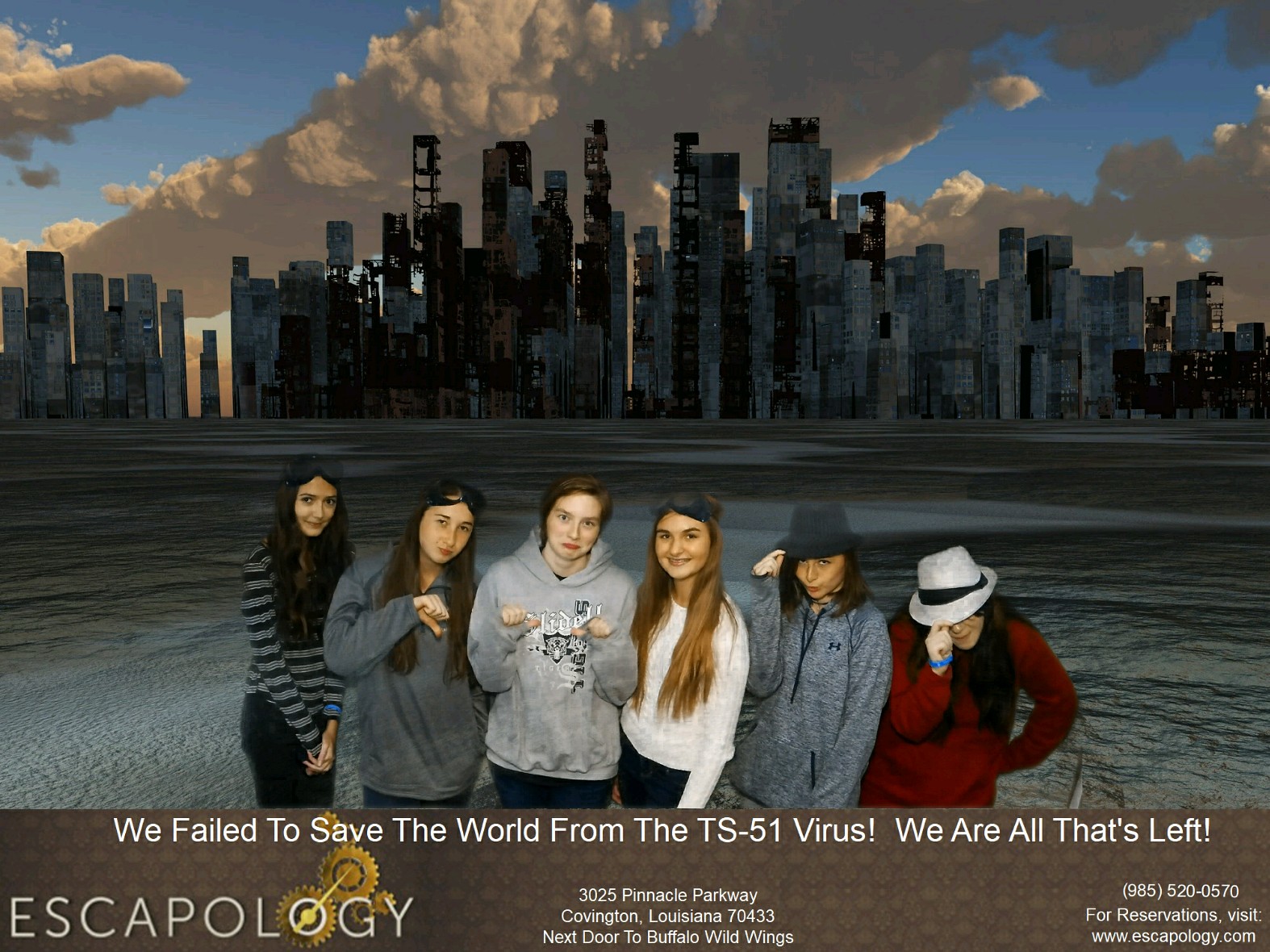In the photo, six girls are posing in front of a desolate New York skyline, which appears ravaged and bombed, suggesting a post-apocalyptic scenario. The landscape where water used to be is now a dry expanse, with nothing but barren ground stretching out. Above the cityscape, clouds hang in a blue sky, adding to the eerie atmosphere. The girls, situated at the bottom of the photo, are making strange faces, with two on the left giving thumbs down. Some of them are equipped with fedoras and safety goggles, enhancing the dystopian theme.

A prominent banner spans the bottom of the image, declaring: "We failed to save the world from the TS-51 virus. We are all that's left." In the bottom left corner, the logo for Escapology is displayed, featuring four interconnected golden gears. The middle of the banner lists the address: 3025 Pinnacle Parkway, Covington, Louisiana, 70433, situated next door to Buffalo Wild Wings. Additional details include a phone number and URL for making reservations, reinforcing that this is an advertisement for an escape room experience that the girls seemingly did not complete successfully.